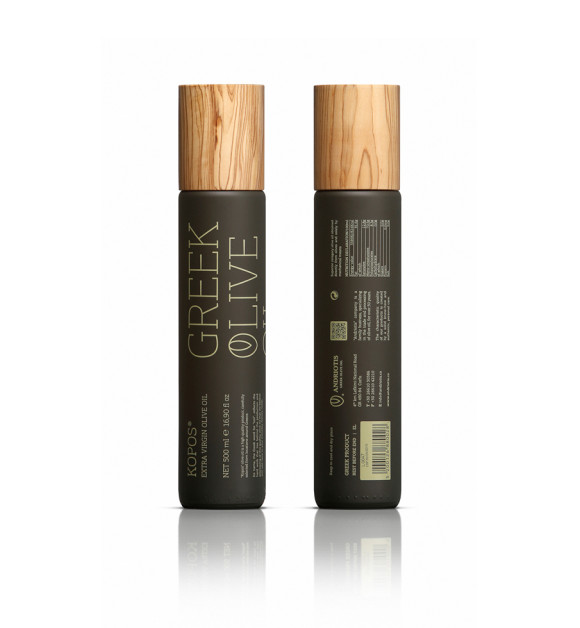The photograph showcases a front-and-back view of a tall, thin bottle of Greek olive oil, prominently labeled "Kopos Extra Virgin Olive Oil." The front view on the left side of the image reveals the distinct design features, including a large wooden screw-on lid and a brown label background. The label displays the text "Greek Olive," with a teardrop-shaped "O" resembling an olive, and further details such as "net 500 milliliters" and "16.9 oz" towards the bottom. The bottle's back view, shown on the right, includes a barcode and nutritional information. The product sits against a white background, and its reflection is visible at the bottom of the image, adding depth to the presentation. The bottle's modern design, with its tube-like shape and wooden cap, lends it an aesthetic often associated with skincare products.